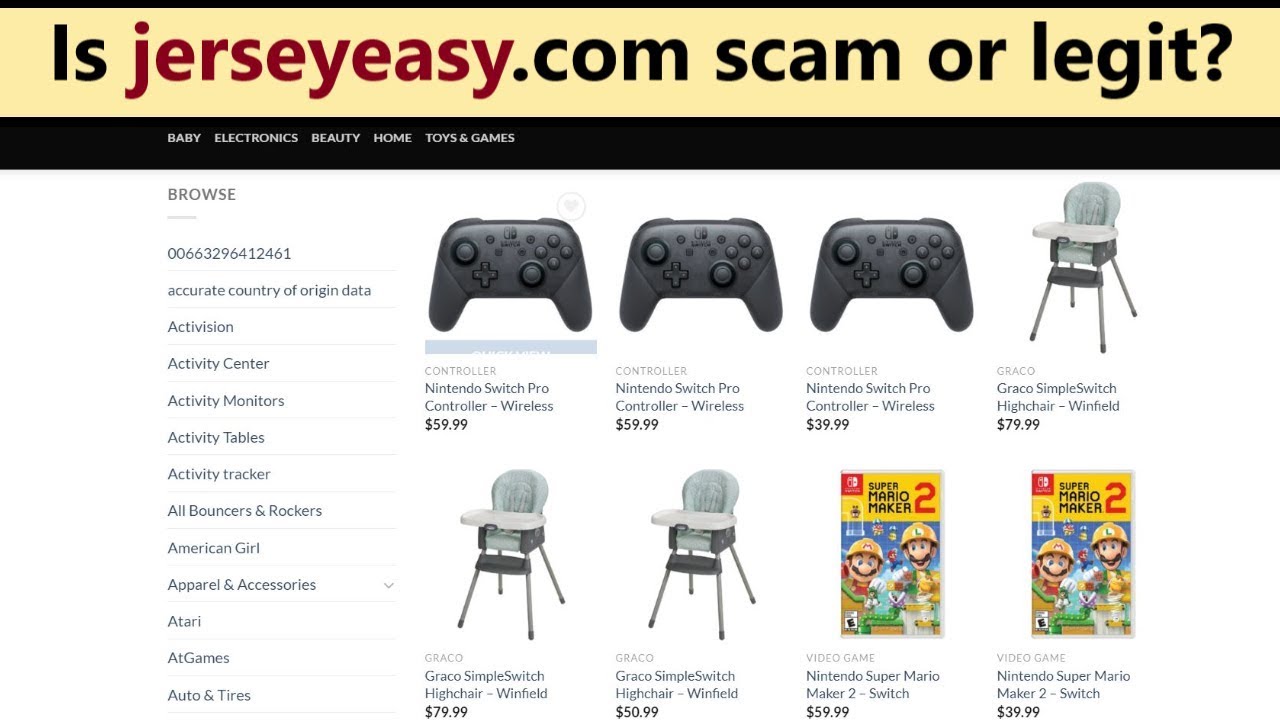Here is the cleaned-up and detailed caption for the image:

---

The screenshot depicts a website with a beige header bar spanning the width of the page, displaying the text "isjerseyeasy.com scammer legit?" in black font. Below the header, there is a black navigation bar with white text, listing categories including "Baby," "Electronics," "Beauty," "Home," and "Toys and Games." Underneath the navigation bar, a vertical menu of links in black font appears on the left side, featuring categories like "Browse," "Accurate Country of Origin," "Date Activision," "Activity Center," "Activity Monitors," "Activity Tables," "Activity Tracker," "Bouncers and Rockers," "American Girl," "Apparels and Accessories," "Atari," "AT Games," and "Auto and Tires."

Positioned to the right of the vertical menu, there are two rows of four item displays each, showcasing products presumably for sale on the website. In the upper left of this section, a "Nintendo Switch Pro Controller" is listed for $59.99. Notably, the screenshot shows this same item listed twice more at the same price of $59.99. However, the last item in this row also displays a "Nintendo Switch Pro Controller" but with an inconsistent price of $39.99, which appears unusual.

---

This detailed caption provides a thorough description of the image, ensuring clarity and an understanding of the website layout and content displayed.